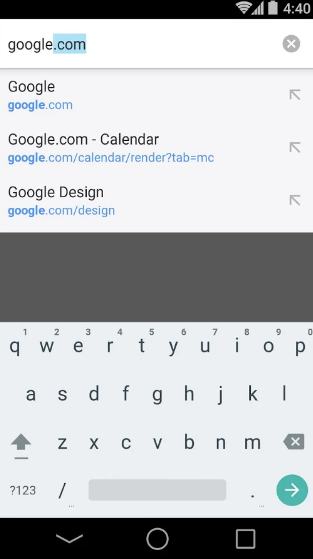This image showcases an older model smartphone, identifiable by its dated design and physical buttons. The device appears to be an Android, as suggested by its interface, although the Wi-Fi is disconnected. The battery is fully charged, and the time displayed is 4:40. The screen shows a Google search tab with "Google.com" entered into the search field, highlighting ".com." The search history reveals multiple entries related to Google, including "Google.com calendar render tab" and "Google design." An on-screen keyboard is visible at the bottom of the screen, displaying a full set of keys similar to those on a computer keyboard. Additionally, icons for a square, circle, and downward arrow are also present at the very bottom of the interface. The font used in the display is standard, contributing to the overall impression of an older generation device. This image appears to be a screenshot taken from the phone.